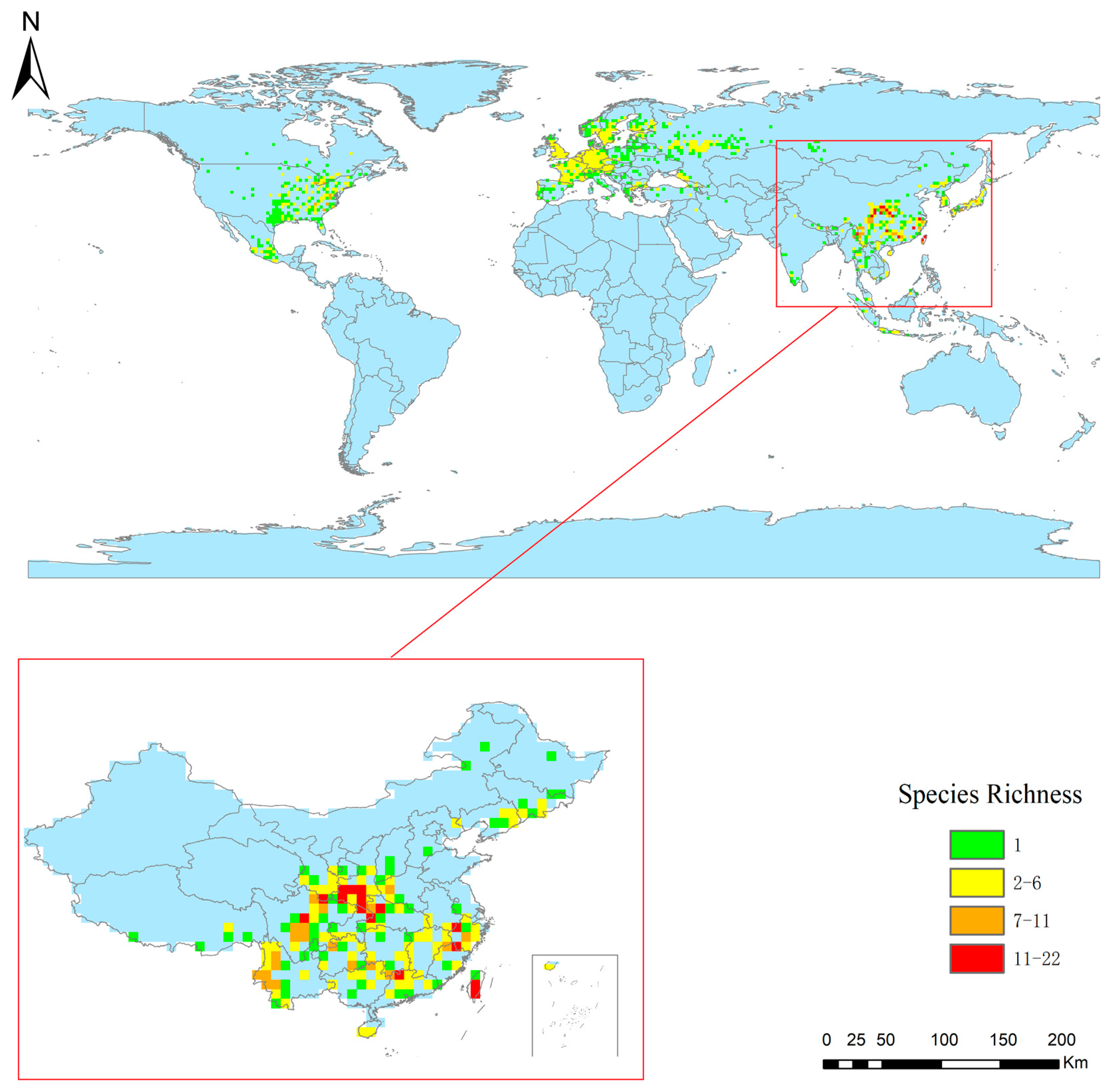This detailed image depicts a flat world map with a vertical rectangular layout and a white background. The map features light blue continents and white oceans, with some areas highlighted in green, yellow, orange, and red, indicating varying levels of species richness. A red box encircles Southeast Asia, with a diagonal line leading to an enlarged inset of this region in the bottom half of the frame. The enlarged section is also color-coded, showing the same range of species richness: green areas represent species richness of 1, yellow areas indicate 2 to 6, orange areas denote 7 to 11, and red areas signify 11 to 22. To the right of the map, a legend explains this color-coding, although it does not specify which species are represented. Overall, this map highlights biodiversity across the globe, with a particular focus on Southeast Asia.